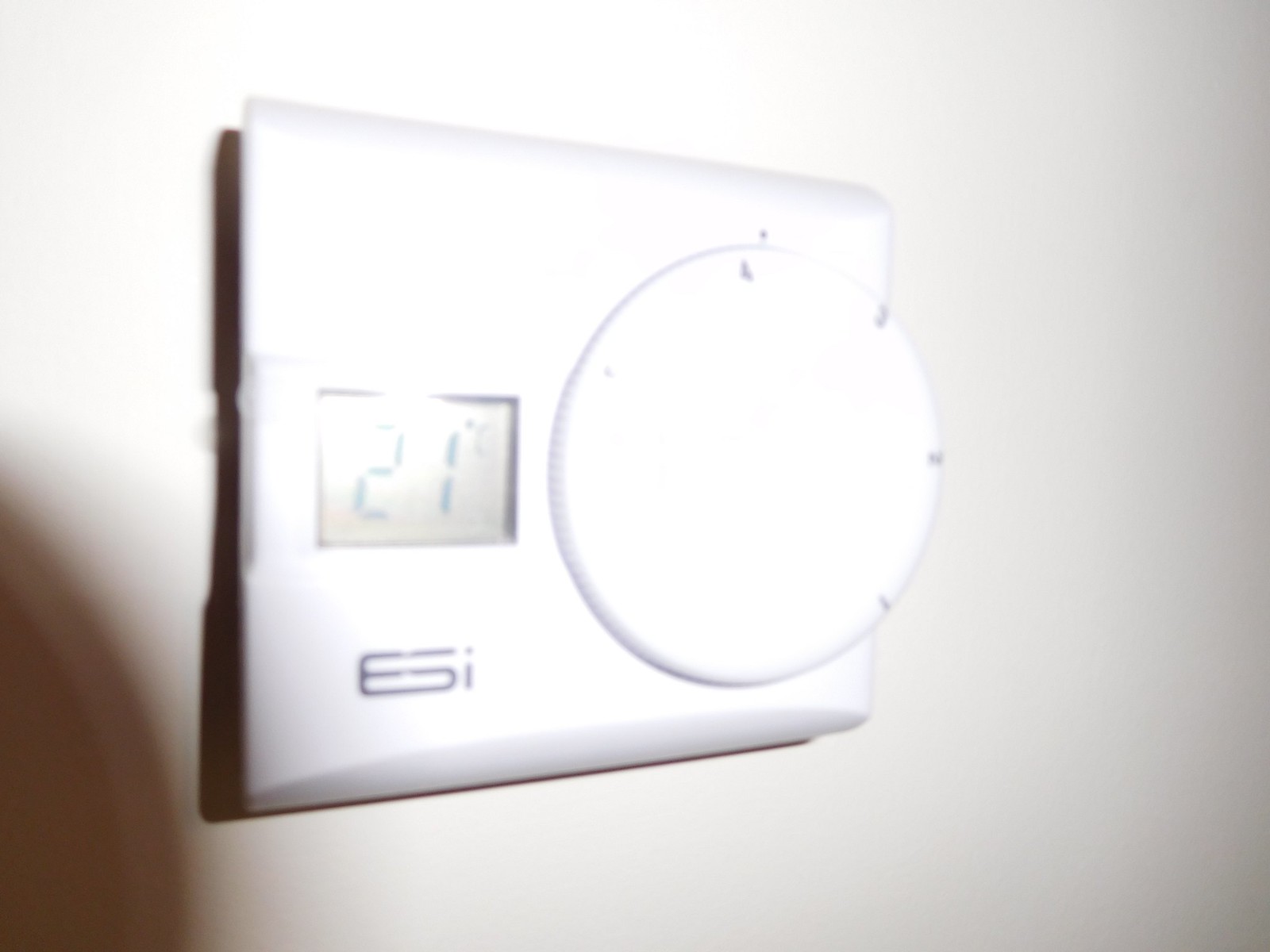The photograph captures a digital thermostat mounted on a white wall, taken with a flash that casts significant glare and reflection. The thermostat is predominantly white, with a prominent circular knob on its right side, likely used to adjust the temperature. The digital display, located in the middle on the left side, shows a temperature reading of 21 degrees Celsius. In the lower left-hand corner of the device, the brand name "ESI" is printed, with "ES" in capital letters. The surface of the dial features several small markings, possibly indicating specific temperature settings or increments. There is a faint shadow on the left side of the thermostat, and a slight shadow resembling a fingertip appears at the bottom left edge of the image. The photograph's overall brightness is intensified by the flash, adding to the glare and reflections on the wall and thermostat.